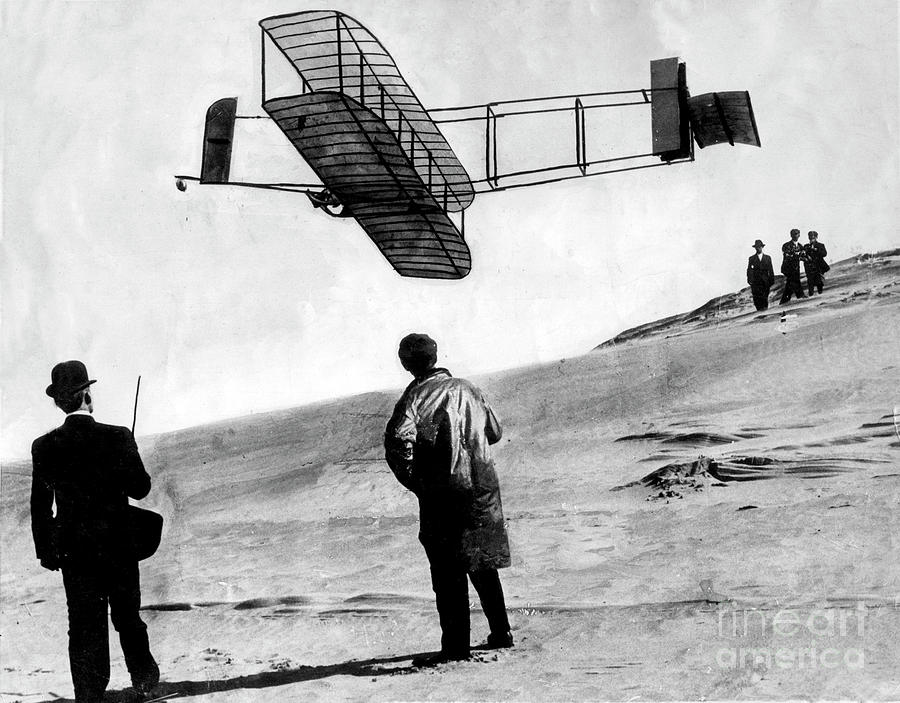This black-and-white drawing, featuring a watermark that reads "Fine Art America" in the bottom right corner, depicts an early aviation scene, likely at Kitty Hawk. The central focus is a primitive glider-type biplane, flying towards the left without any visible propellers but equipped with a long rudder and gauzy wings. On the left side of the image, in the foreground, two men with their backs turned to the viewer observe the plane. The man in the left corner is dressed in a black suit and bowler hat, holding an object resembling an antenna. Beside him, another man is bareheaded and outfitted in outdoor attire, such as a long coat. Further up, three additional figures stand atop a hill or mountain, similarly dressed, one notably in a bowler hat, all watching the aircraft. The scene underscores the pioneering days of aviation, capturing both the curiosity and the rudimentary technology of the era.